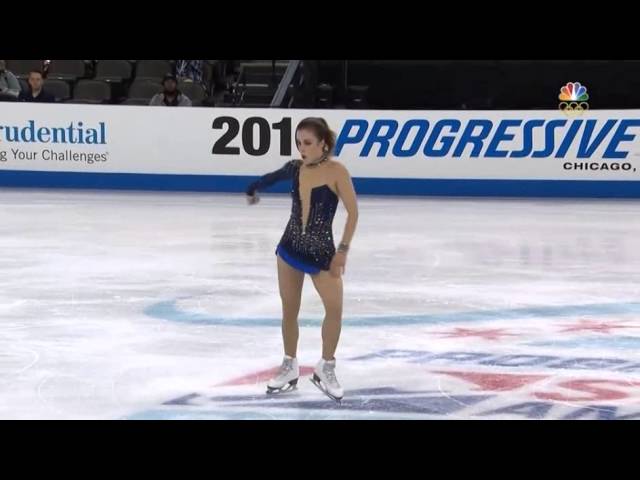In this image, an ice skater is captured mid-performance in an indoor arena, likely during a competitive event, potentially the Olympics, as suggested by the Olympic rings and NBC peacock logo in the upper right corner. The skater, positioned at the center of the ice rink, is dressed in a striking black skating outfit with one long sleeve and sparkling elements, including a bit of blue at the bottom of her short skirt. She also wears white figure skates and a sparkly wrist bracelet on her left wrist, adding to her elegant appearance. Her serious expression and downward gaze are highlighted as she performs a twisty move. The ice rink itself is white with blue and red markings, bearing some inscriptions, while the barrier surrounding the rink is predominantly white with blue at the bottom, featuring advertisements for Progressive and Prudential, and partially visible text that reads "Progressive" and "Chicago". Behind the barrier, a darkened area reveals a few spectators, engulfing the scene in a competitive ambiance.